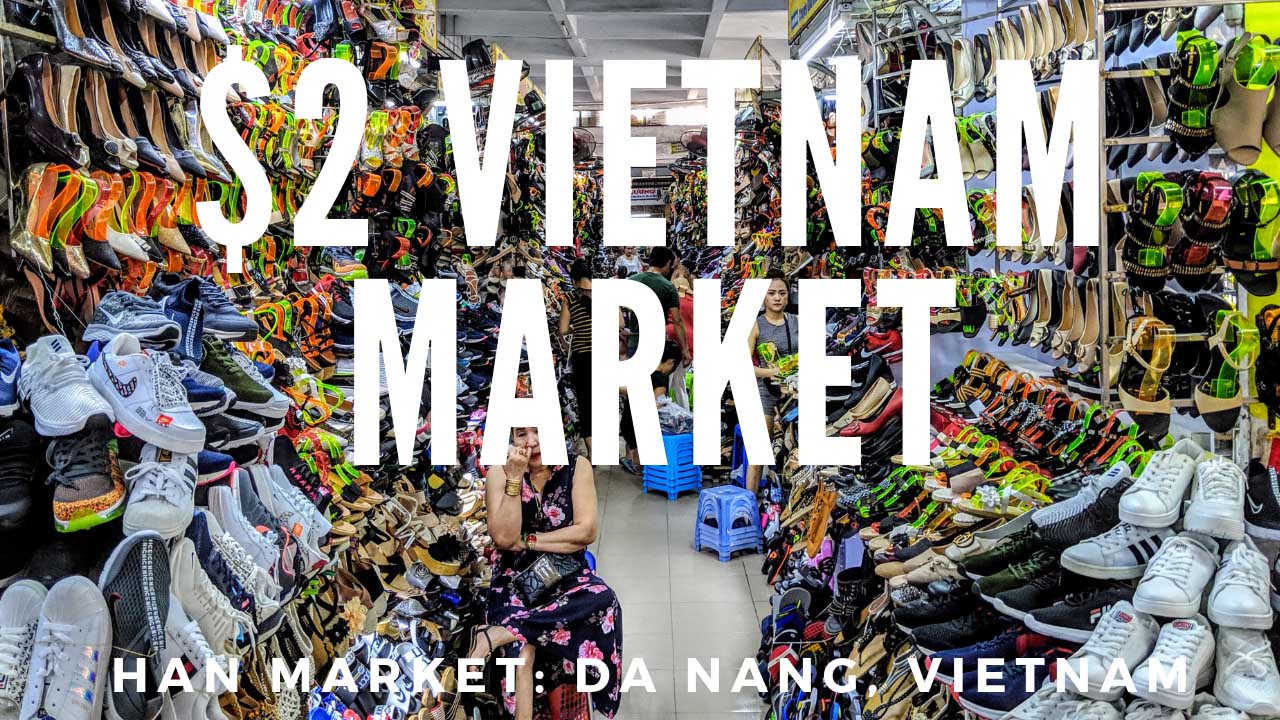The image depicts a cluttered and vibrant storefront in Vietnam, specifically the Han Market in Da Nang. The shop is crammed with a diverse array of shoes, including sneakers and high-heeled women's shoes, displayed from floor to ceiling on tall shelves that line both sides of a narrow aisle. The shoes are in a multitude of colors—green, black, white, and blue, among others. There is an air of bustling activity with several shoppers in the background, and in the center of the aisle, a woman sits on one of the blue stools, looking somewhat exhausted. The scene is topped off with large, bold white text reading "$2 Vietnam Market," prominent in the center of the image, with "Han Market, Da Nang, Vietnam" written at the bottom.